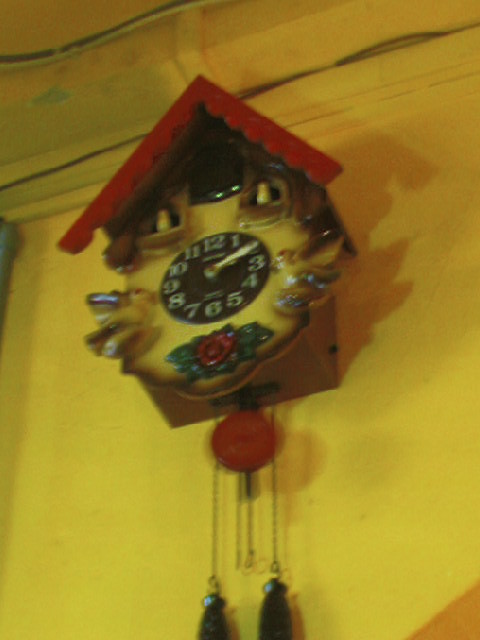This image features a traditional Bavarian cuckoo clock, though the image quality is somewhat blurry. The clock is predominantly yellow and is mounted against a matching yellow wall. The clock face stands out with its dark brown color and white numerals from 12 to 3, arranged in the usual clockwise fashion. The roof of the cuckoo clock is a vibrant red, as is its pendulum. Hanging below the clock, there are dark brown, pine cone-shaped weights, which are crucial for the clock's mechanism. Additionally, at the top of the clock, two small objects protrude, possibly decorative elements. The clock also features intricate designs including flowers and a bird, though the details are not completely clear due to the blur in the image. The background includes a glimpse of a yellow ceiling.